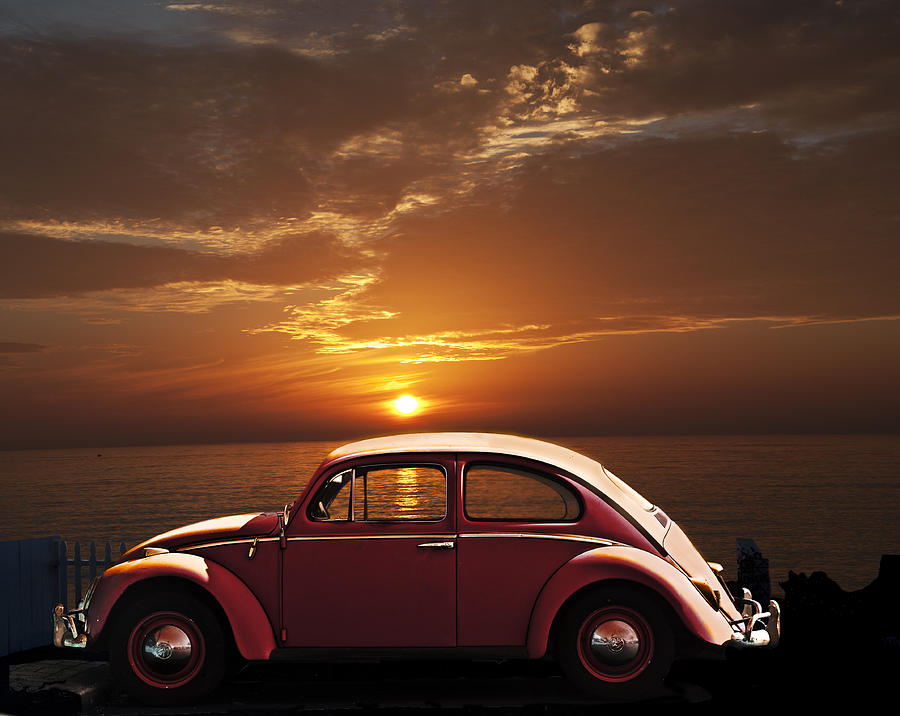A vintage red Volkswagen Beetle is parked on a road by the ocean, basking in the glow of an orange sunset. The car, with its classic rounded shape, silver bumpers, hubcaps, and a back spare tire, is vividly detailed against a breathtaking backdrop. The horizon showcases the sun, a large glowing yellow orb casting an orange trail across the calm, tannish waters. The sky is a dramatic mix of dark gray, brown, and orange clouds with streaks of white and hints of blue peeking through. The scene is divided by a fence, separating the bright and serene ocean view from the iconic vehicle. The sun’s rays illuminate parts of the car, enhancing its deep red color and making it a poignant highlight of this beautifully composed, atmospheric image.